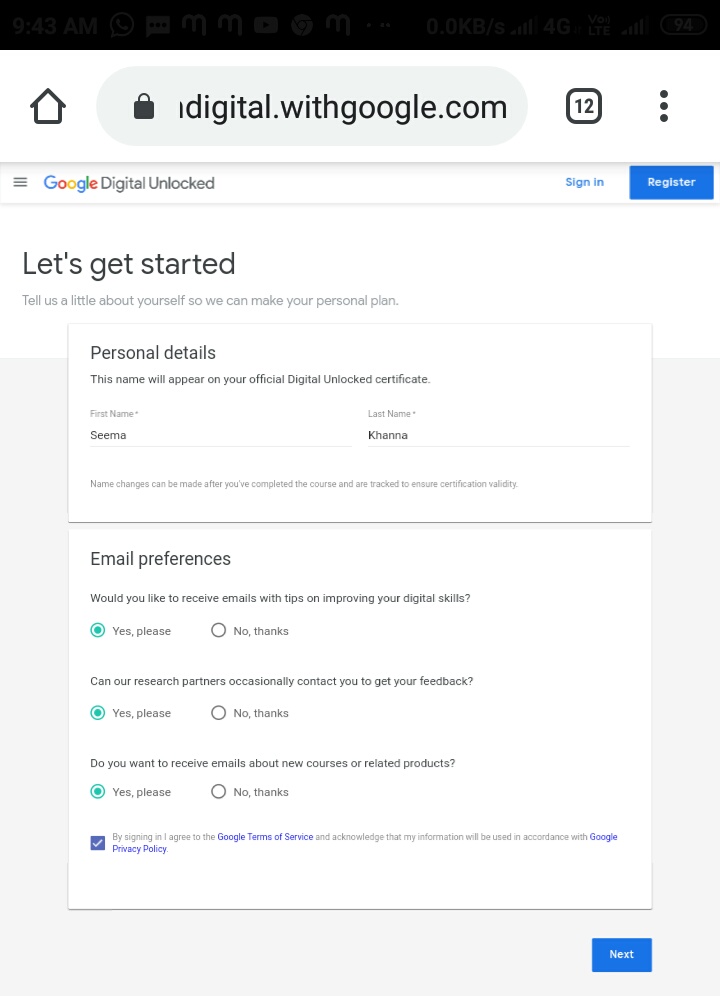The image displays a webpage interface for Google's "Digital Unlocked" initiative. At the top, there is a black navigation bar, followed by a white section. On the left side of this section, a house icon and a lock icon are accompanied by the text "digital.withgoogle.com." 

Immediately below, a black box features the digits "1" and "2," while three vertical black dots sit next to it. Adjacent to these, three horizontal black lines are visible. The Google Digital Unlocked logo is prominently displayed with "Google" in its iconic colors: blue, red, yellow, blue, green, and red. To the right of the logo, there is a small "Sign In" link in blue text, accompanied by a blue "Register" button with white text.

Further down the page, a heading in black text reads, "Let's get started," followed by a smaller subheading, "Tell us a little about yourself so we can make your personal plan." Centered beneath this text, a white box labeled "Personal Details" appears, with an additional note about the name appearing on the official Digital Unlocked certificate. The text "Digital Unlocked" is capitalized for emphasis. 

Below this, fields for "First Name" and "Last Name" are filled out with "SEEMA" and "KHANNA," respectively. A disclaimer in small font indicates that name changes can be made after course completion to ensure certification validity.

The page also includes an "Email Preferences" section with options asking if the user would like to receive emails on improving digital skills (with "Yes, please" selected and turned green), if research partners can contact them for feedback (also selected as "Yes"), and if they wish to receive updates about new courses or products ("Yes, please" is selected).

At the bottom of the form, a blue box with a white check mark is followed by a notice in tiny font that reads, "By signing in, I agree to the Google Terms of Service and acknowledge that my information will be used in accordance with Google Privacy Policy." The terms "Google Terms of Service" and "Google Privacy Policy" are highlighted in blue text. Finally, on the bottom right corner, there is a blue "Next" button with white text.